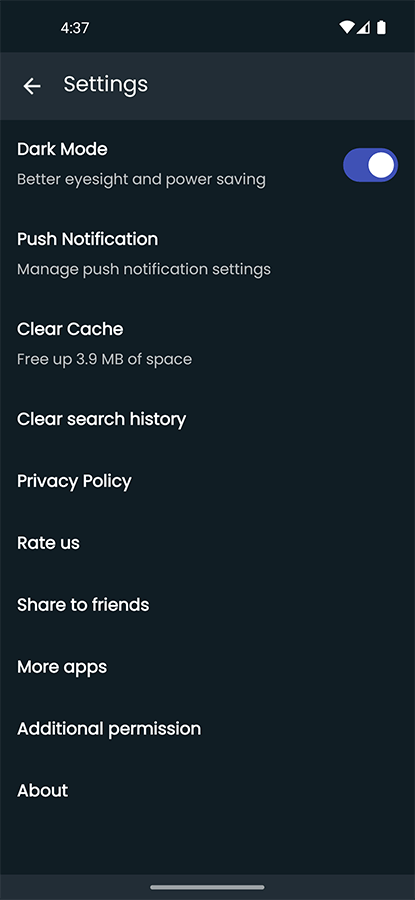This image is a phone screenshot displaying a settings menu with a dark blue rectangular background. At the top left, there is the number "437" in white text. On the top right, there are three white icons: a fully connected Wi-Fi symbol, a partially filled signal strength icon, and a fully charged battery icon.

Below this, the menu includes an arrow pointing to the left followed by the word "Settings" in white text. This section is highlighted with a bluish-gray rectangle, which the same background color is used again underneath for consistency.

The menu options are listed in white text against the dark background. The first option is "Dark Mode," which is followed by the phrases "Better eyesight" and "Power saving." There is a blue toggle switch next to this option, indicating that dark mode is turned on. 

The next option is "Push Notifications" with a subtitle "Manage push notification settings." This is followed by "Clear Cache" with "Free up 3.9 megabytes of space," "Clear Search History," "Privacy Policy," "Rate Us," "Share to Friends," "More Apps," "Additional Permission," and "About."

At the bottom right of the screen, there is a section with the same background color as the top "Settings" rectangle, separated by a gray line running horizontally across the center.